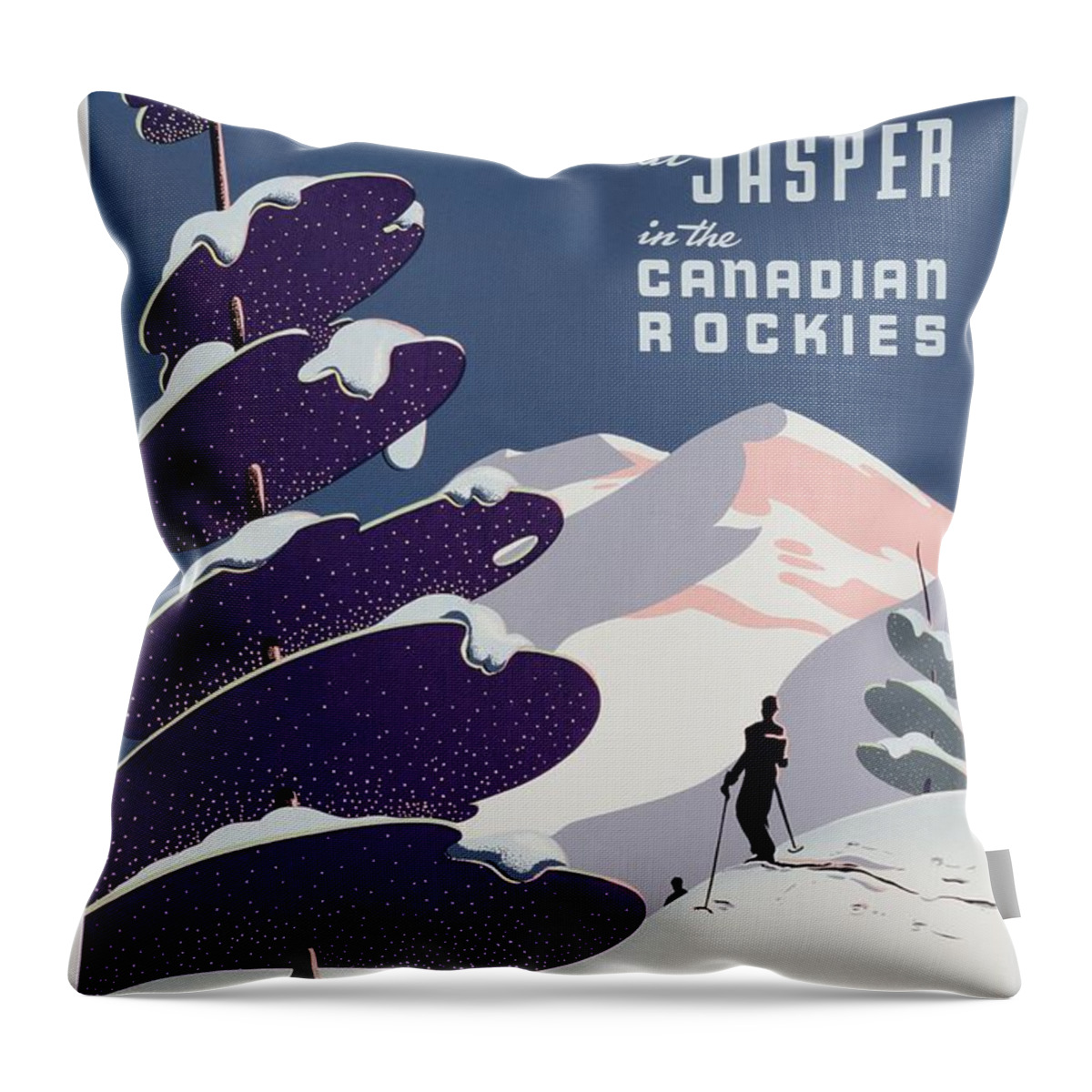The image is a detailed mock-up of a commemorative pillow designed for the Jasper Ski Resort in the Canadian Rockies. The square pillow, depicted against a plain white background without a border or frame, features a detailed and stylized graphic design. 

On the left side is a unique and abstract representation of a conifer tree. The tree is made up of five circular sections resembling mushrooms on a skewer, with each section colored purple with yellow spots and topped with layers of snow, presenting a whimsical winter aesthetic. 

To the right of this tree, the eye is drawn to a stylized mountain range. The two prominent peaks are rendered in shades of white, gray, and light pink, creating a sense of depth with their salmon-colored shadows blending to the right. 

In the lower left corner, adding a dynamic touch to the scene, is the black silhouette of a skier poised on a small hill. The skier appears to be captured mid-motion, with ski poles extending both forward and behind, suggesting movement against the softly shadowed gray snow.

Above this tranquil winter scene, the pillow proudly displays the text "Jasper" in light blue, capitalized stylized letters set against a grayish dark blue sky. Below Jasper, in a script font, it reads "INDA," followed by "CANADIAN ROCKIES" in all caps. The overall artwork combines modern artistic elements with a charming, playful interpretation of a winter landscape, making it a fitting tribute to the beauty and spirit of the Jasper Ski Resort.